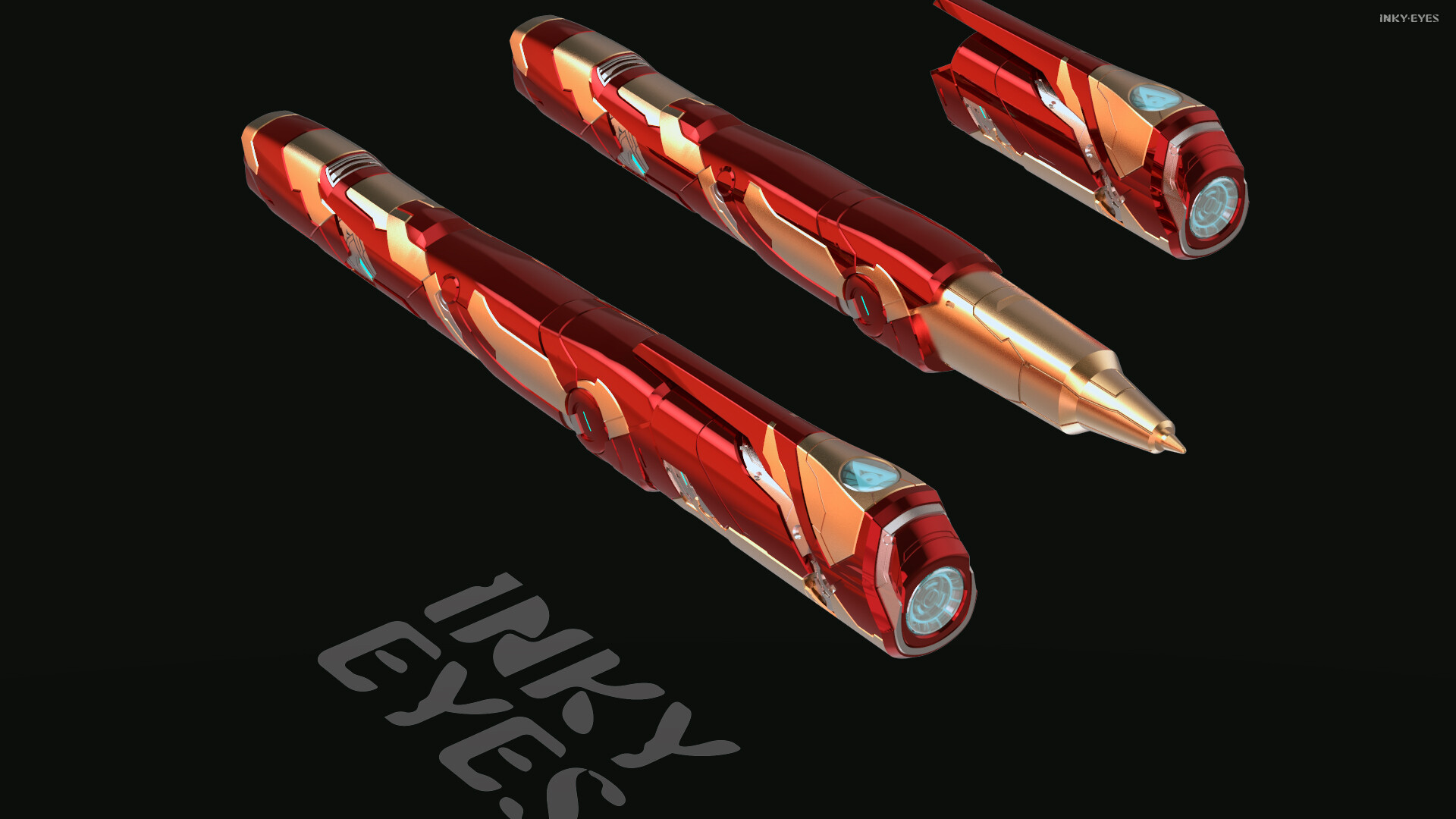Against a stark black background, the image showcases three red and gold shiny objects: two flashlights and one pen. The upper left corner features a long, ornate flashlight with a light at its tip, extending diagonally to the lower middle of the frame. Adjacent to it in the upper middle of the image is a pen, also red and gold, with its tip pointing towards the lower right corner. In the upper right quadrant, there is a stubby flashlight, directed similarly towards the bottom right. Near the bottom, gray text diagonally spans from left to right, reading "INKY EYES." The composition emphasizes the metallic sheen and vivid colors of the objects, contrasting sharply with the dark background.